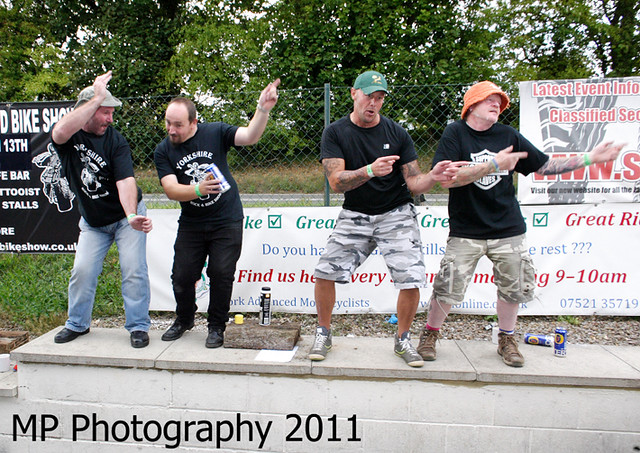In the image, taken by MP Photography in 2011, four males of varying ages are captured goofily dancing on top of a brick ledge outdoors, possibly in the middle of the day. They are arranged centrally within the frame, all pointing to the left with both fingers. 

From left to right, the first man is wearing a lighter green hat, a black T-shirt, light blue jeans, and black shoes, appearing to be in a jovial dancing pose. The second man, slightly balding with brown hair, a mustache, and a beard, is dressed in black pants, black shoes, and a black shirt with a white logo. 

Next, the third man, aged around 30s or 40s, wears a black shirt, green cap, camo shorts, and sneakers. Finally, the fourth man seems older, possibly in his 50s, and he is adorned with an orange hat, a black T-shirt, camo shorts, and brown boots. 

Behind them, there is a fence embellished with various posters and signs, adding to the vibrant outdoor setting. The backdrop also includes some greenery with trees and shrubs, enhancing the lively and natural ambiance of the scene.